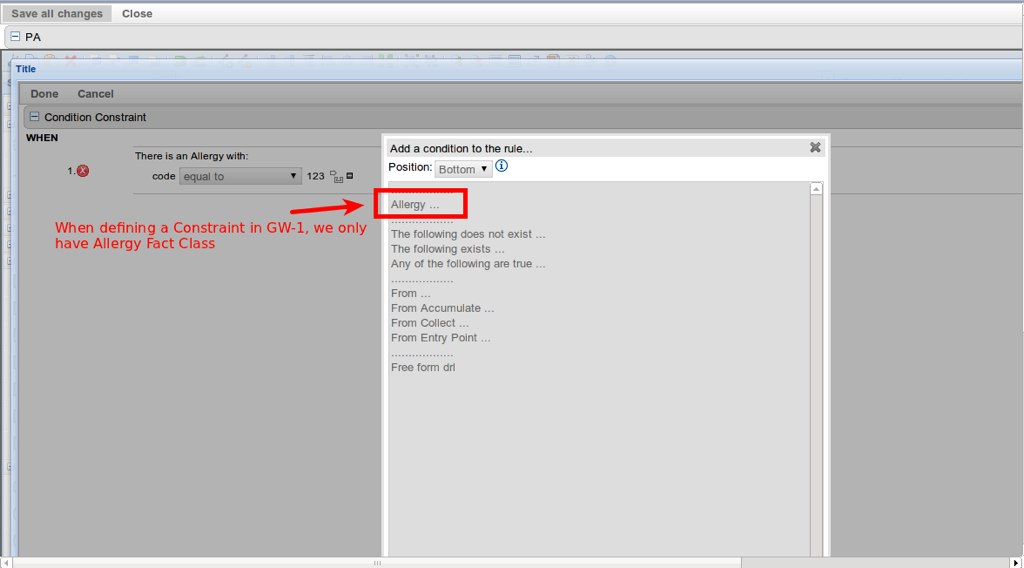The screenshot displays a software program window with a predominantly gray and white interface. At the center is a gray pop-up box titled "Add a condition to the rule." Within this box, several lines of text are listed: "Position" followed by a dropdown arrow and an eye icon for additional information. Subsequent listings include "Allergy," "The following does not exist," and "Any of the following are true." Below these lines, terms such as "from," "from accumulate," "from collect," and "from entry point" are mentioned, terminating in another set of dots. There's a line marked "Free form DRL."

On the left side of the window, red text states, "When defining a constraint in GW-1, we only have allergy fact class," accompanied by a red arrow pointing to the word "Allergy" and a red-outlined box emphasizing it. The background is consistently gray, with some sections difficult to read due to unfocused text. The overall appearance suggests use in a training context or instructional manual for the software.